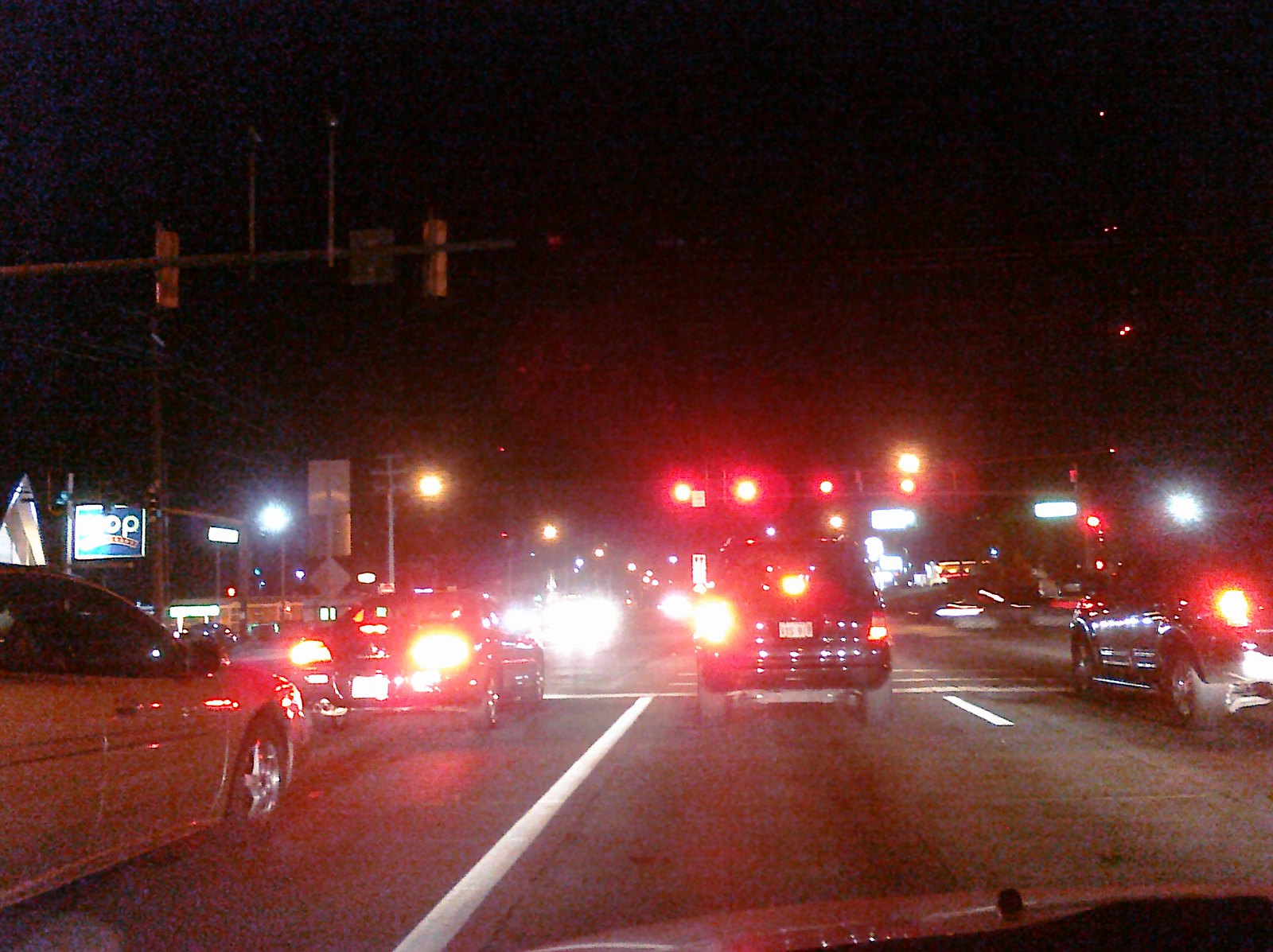In this nighttime cityscape, we find ourselves positioned in the driver's seat of a car, halted at a red stoplight on a busy street. The dimly lit scene is dominated by the glow of streetlights and the unmistakable red of the overhead stoplights. Directly in front of our car, a single vehicle waits, separated by a noticeable gap. The traffic is more congested to our left, where two cars line up side by side, while a lone car occupies the lane to our right. Amidst the shadows and limited visibility of the night, an IHOP restaurant punctuates the scene on the left-hand side, its sign clearly illuminated by an external light, serving as a distinctive landmark in this urban setting.